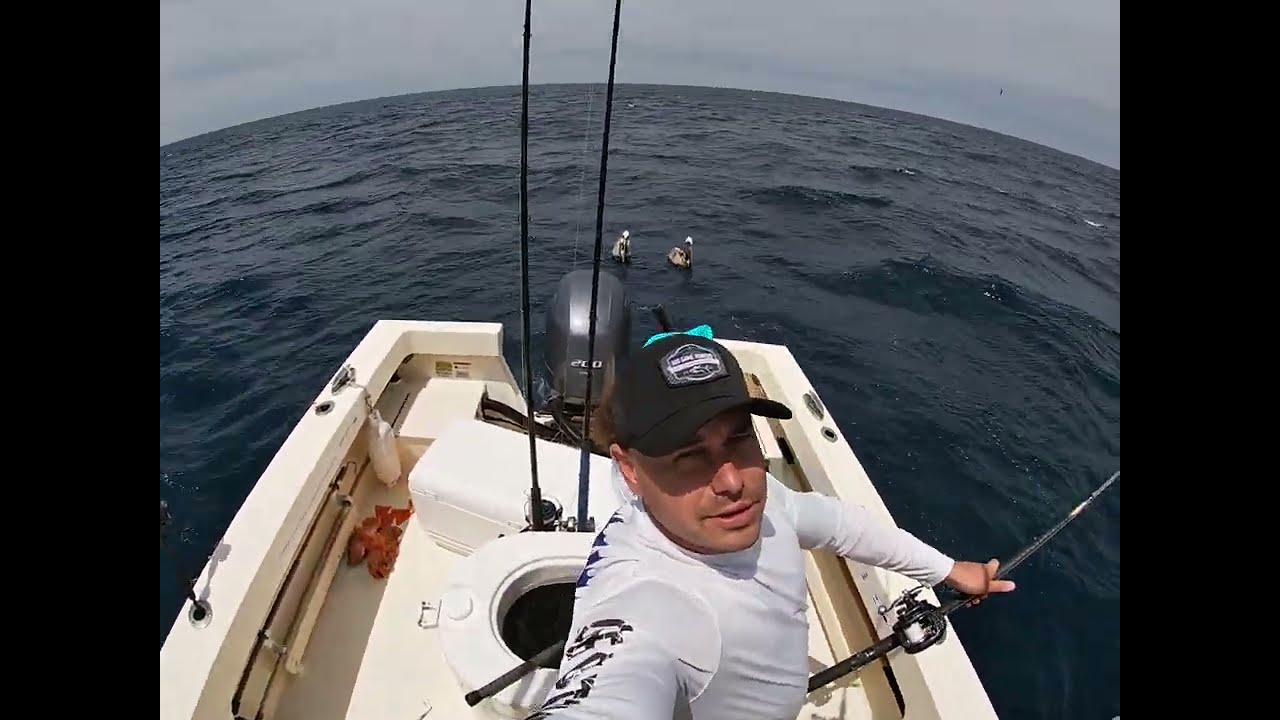In this detailed image, a man is captured on a small white boat, which has an engine mounted on its back. The man, wearing a black hat and a long-sleeve white rash guard material shirt, is taking a selfie with his right hand while holding a fishing rod over the edge of the boat with his left hand. The boat, devoid of any roof, sits in the vast expanse of water with no land in sight, under a cloudy midday sky. The photo's lens creates a dramatic curvature of the water, prominently featuring a curved horizon line. In the background, a couple of ducks or pelicans can be seen swimming in the ocean, adding a touch of wildlife to the serene fishing scene. Various fishing gear and possibly some bait or fish are visible inside the small rectangular craft.